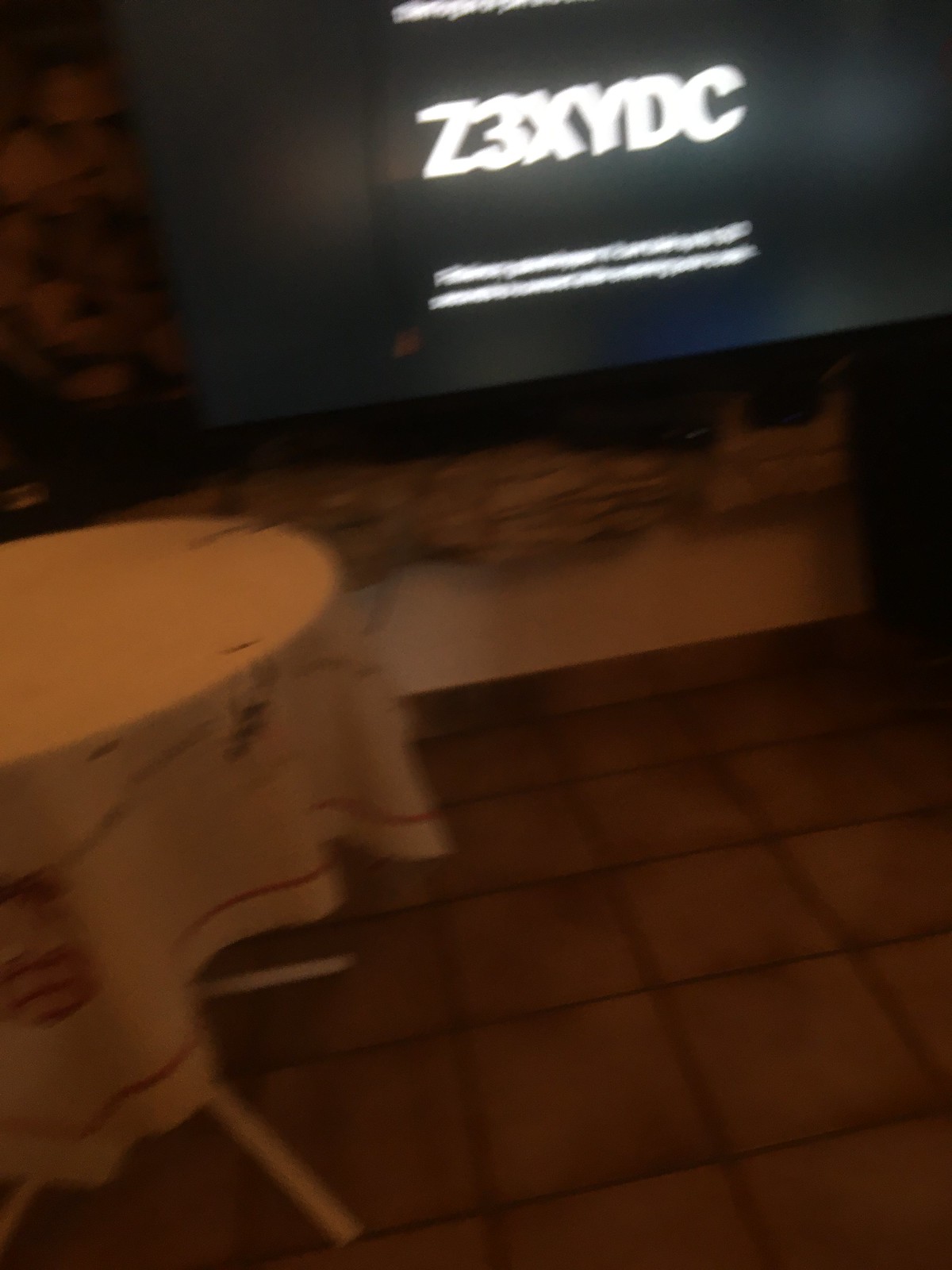This photograph portrays a somewhat blurry, dimly lit dining room or café corner, featuring a small, circular table with thin, slanting legs, adorned in a white tablecloth with an embroidered decorative border of green leaves and red lines. The table stands on a dark chocolate brown tiled floor, each small square tile separated by matching dark brown grout. Adjacent to this table, mounted on a wall with a tan and brown stone-like backing, is a television screen displaying a code "73XYDC" in white capital letters on a black background, accompanied by two unreadable lines of text below it. Below the stone wall is an extended strip of a white wall, and a small sliver of brown wood can be seen under the TV. The TV screen itself appears tilted upwards towards the right by about 20 degrees, adding to the image's overall sense of unsteady composition.